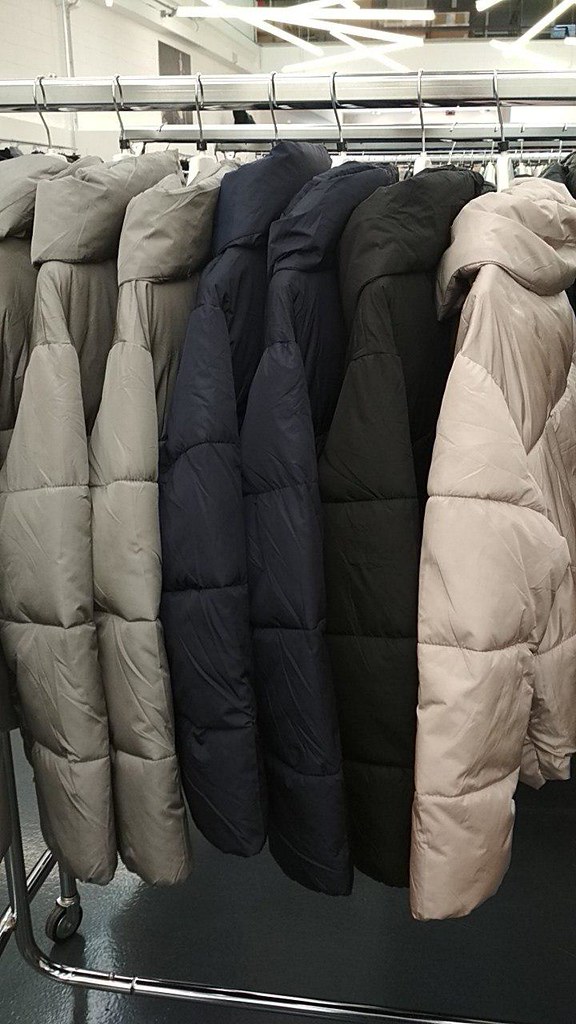The image showcases a digital photograph taken inside what appears to be a department store or a storage area for a department store. The upper left portion of the photo features a very bright white wall, accentuated by modern, skinny rectangular lights that are suspended from the ceiling, emitting an extremely bright white illumination. 

The bottom of the photograph reveals a nicely polished bright gray floor, indicative of recent maintenance. The central focus is a metal rack on black wheels that holds coats on sturdy, white plastic hangers. The hanger rod itself is made of silver metal. 

From left to right, the first three coats are gray and puffy, each featuring a hood and considerable length. Following the gray coats, there are two dark blue coats. The next color appears to be almost a burgundy hue, and finally, the rack ends with a lighter, cream-slash-beige colored coat on the far right.

Although some color descriptions differ slightly, the image prominently displays a selection of long, hooded, puffy coats organized by color on a single metal rack.